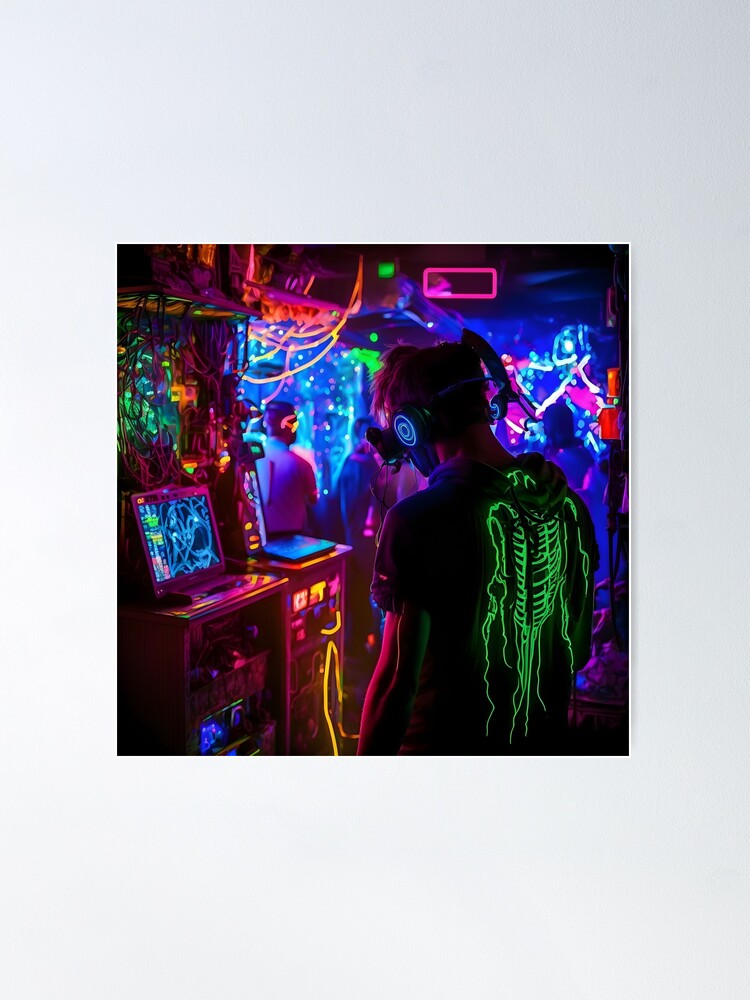The image depicts the interior of a dark, neon-lit room that resembles an old video arcade or dance club. The photograph is vertically rectangular with a light gray border, but the central image is square, filled with a kaleidoscope of fluorescent colors such as pink, orange, yellow, blue, red, and green, all against a predominantly black background. In the forefront, just to the right of center, stands a man with his back to the camera, wearing a dark-colored t-shirt that features a glowing green design—possibly of a monster, a fish, or something resembling a skeleton—illuminated by black light. He appears to be wearing headphones and is facing a setup resembling arcade or musical equipment, including what looks like a monitor or laptop on a stand. Above him, yellow and pink lines hang from the ceiling, adding to the vibrant atmosphere. To the upper left, there's a green object visible in the background, while the far end of the room features more people either dancing or standing, bathed in hues of blue and purple. The entire scene is awash with myriad neon and fluorescent lights, giving the impression of a lively, energetic space filled with electronic entertainment.